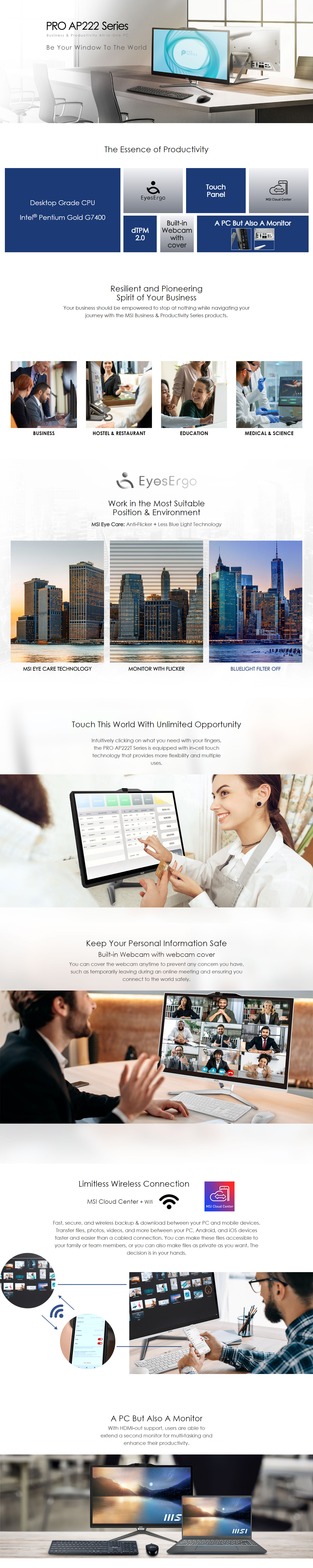Here's a refined and detailed caption:

"A comprehensive, full-length screenshot of a website showcases the entire page from top to bottom, capturing the full scope without the need for scrolling. At the very top, an expansive banner image depicts an office setting with a desk and a computer monitor. Superimposed over the image is the text 'Pro AP 222 Series.' Just beneath, the website transitions to a clean, white background with the tagline, 'This is the essence of productivity.' Following this, a section featuring a visually striking grid layout appears, composed of seven blocks — three in gray and four in blue — arranged in varying sizes. Further down the page, another text section reads 'Resilient and Pioneering,' though the text appears slightly distorted and difficult to read."